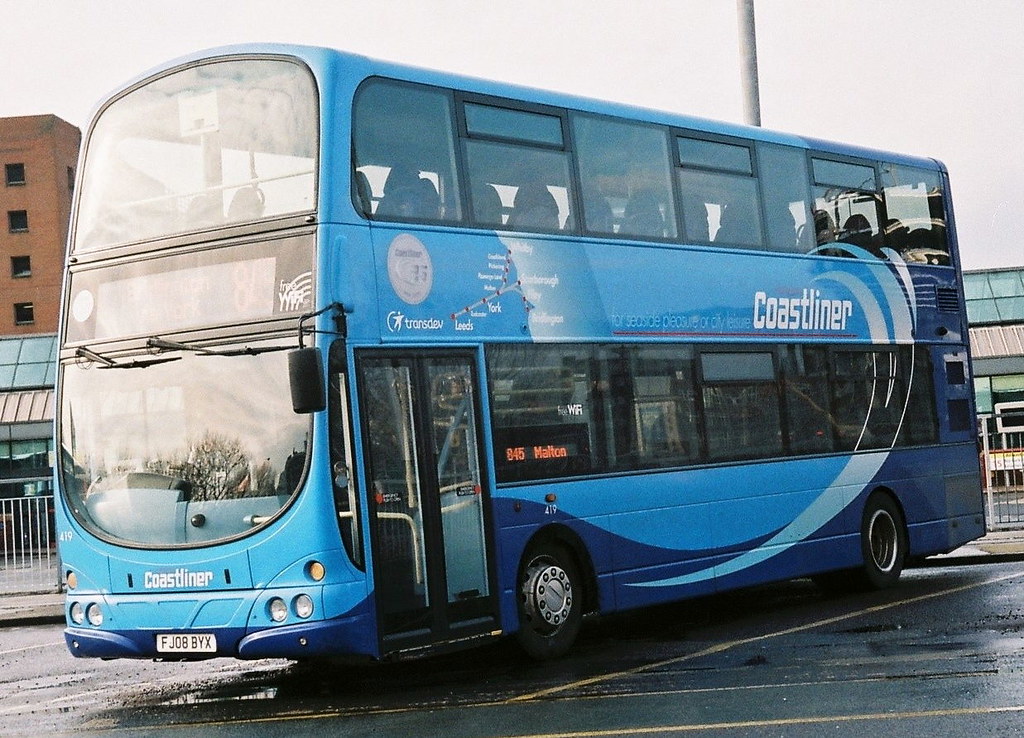In an outdoor setting, there is a distinct blue double-decker bus prominently displayed in a parking lot. The bus features varying shades of bright and dark blue. "COASTLINER" is written in bold white letters on both the side and the front. It also showcases the label "045 Malton" along with a notice about Wi-Fi availability on the top. The license plate reads FGO8BYX. Although no passengers are visible on this stationary bus, it has both upper and lower seating areas, discernable through its windows. A double door is located at the front on the lower level. Surrounding the bus, the pavement shows the clear markings of the parking lot. In the background, a multi-story building with a combination of brick and glass, complete with an awning, stands to the left. Further back, another building with glass skylights or a rooftop glass structure adds to the scene.